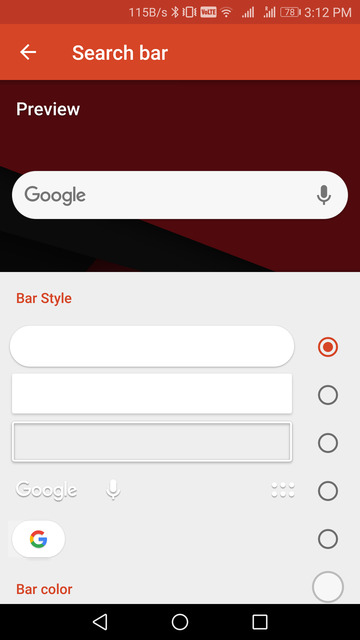A vertically oriented screenshot from a smartphone displays several interface elements. At the top, a thin, dark red rectangle spans horizontally, indicating a status bar. Inside it, icons and information are visible: the text "11 5BSs," a Bluetooth symbol, a video icon, Wi-Fi indication, signal strength, battery life showing at 70%, and the time "3:12 PM" aligned to the far right.

Beneath this, a slightly lighter yet thicker red rectangle is present, featuring a left-pointing white arrow and the text "search bar" in white. The primary background is a deep crimson red that darkens to near-black towards the bottom left corner. In the upper left, the word "Preview" is discernible.

Below this header, a Google search bar is prominently displayed with a right-aligned microphone icon. Further down, a gray box contains various customization options. It states "bar style" in orange, accompanied by a rounded white search box, a rectangular white search box with square corners, and another gray box. Multiple selectable circles are present, with the first one highlighted in orange. The options are accompanied by the text "Google" and include a microphone icon and a grid icon, as well as a Google logo. Additional text reads "bar color," addressing further customization.

At the bottom of the screenshot, a black rectangular strip features interface controls: a leftward-pointing arrow on the left side, a centered circle, and a square on the right.